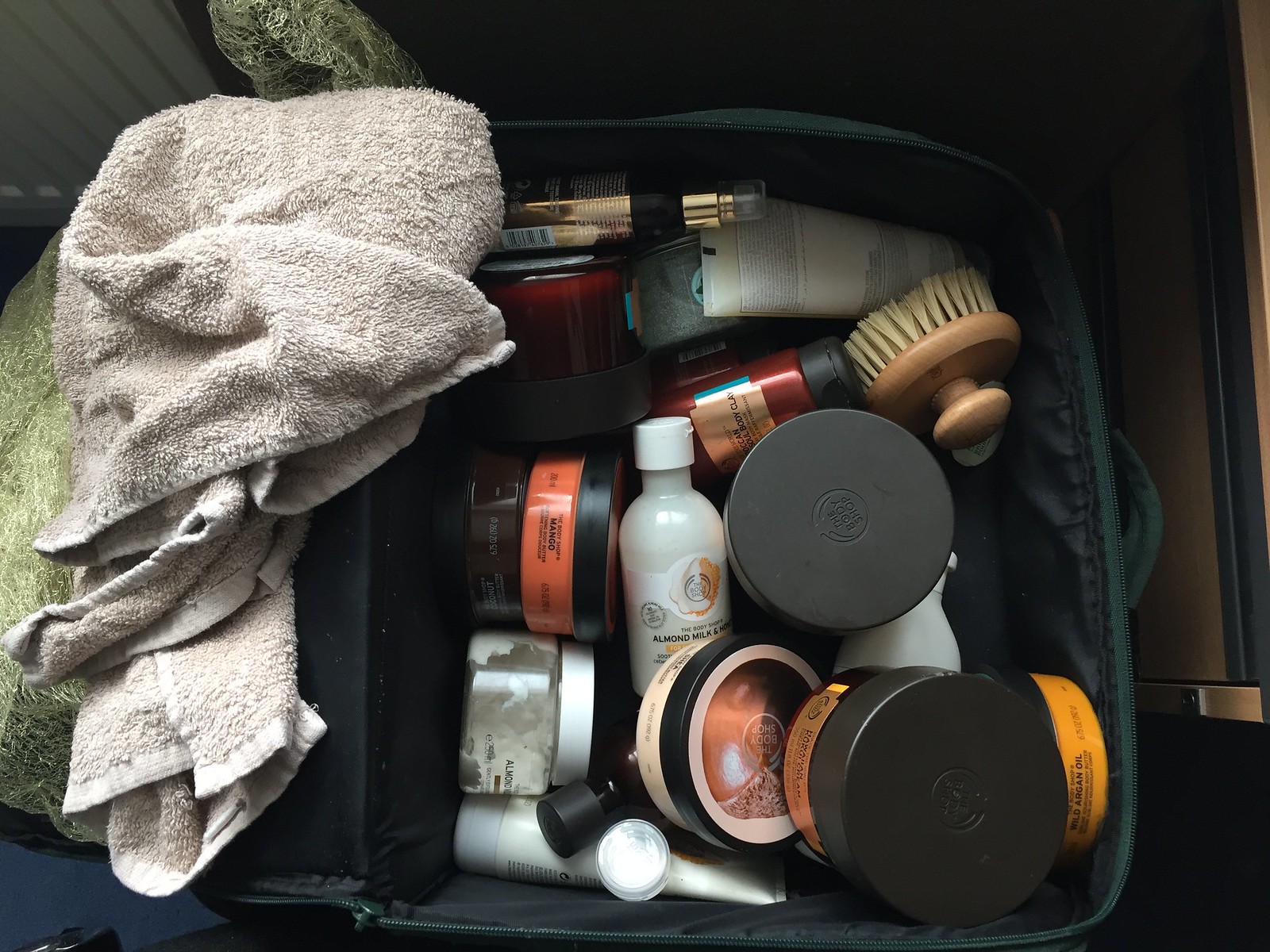This image depicts a spacious cosmetic case filled with an array of beauty products, all haphazardly arranged. To the left of the case, a tan towel is bunched up, partially covering an orange plastic shower cap meant to keep hair dry during showers or baths. Beneath this towel lies another fabric item, either another towel or blanket, though its exact nature is unclear. Adjacent to these items is a radiator.

The main focus of the picture is the open cosmetic case, brimming with an assortment of products, predominantly from The Body Shop. Visible items include an "Almond Milk & Honey" product, along with various bottles of argan oil and a mango-scented item. There is a brown-handled nail brush with yellow bristles, used for scrubbing fingernails.

The products vary in size and type: some are body clays in small canisters, others are lotions in long-neck, squeezy bottles, and some are contained in spray bottles. A few items are housed in tiny travel vials. The containers come in various colors—white, orange, dark red, and gray—adding a splash of color to the green cosmetic case. The case is fully open, allowing a clear view of its diverse contents.